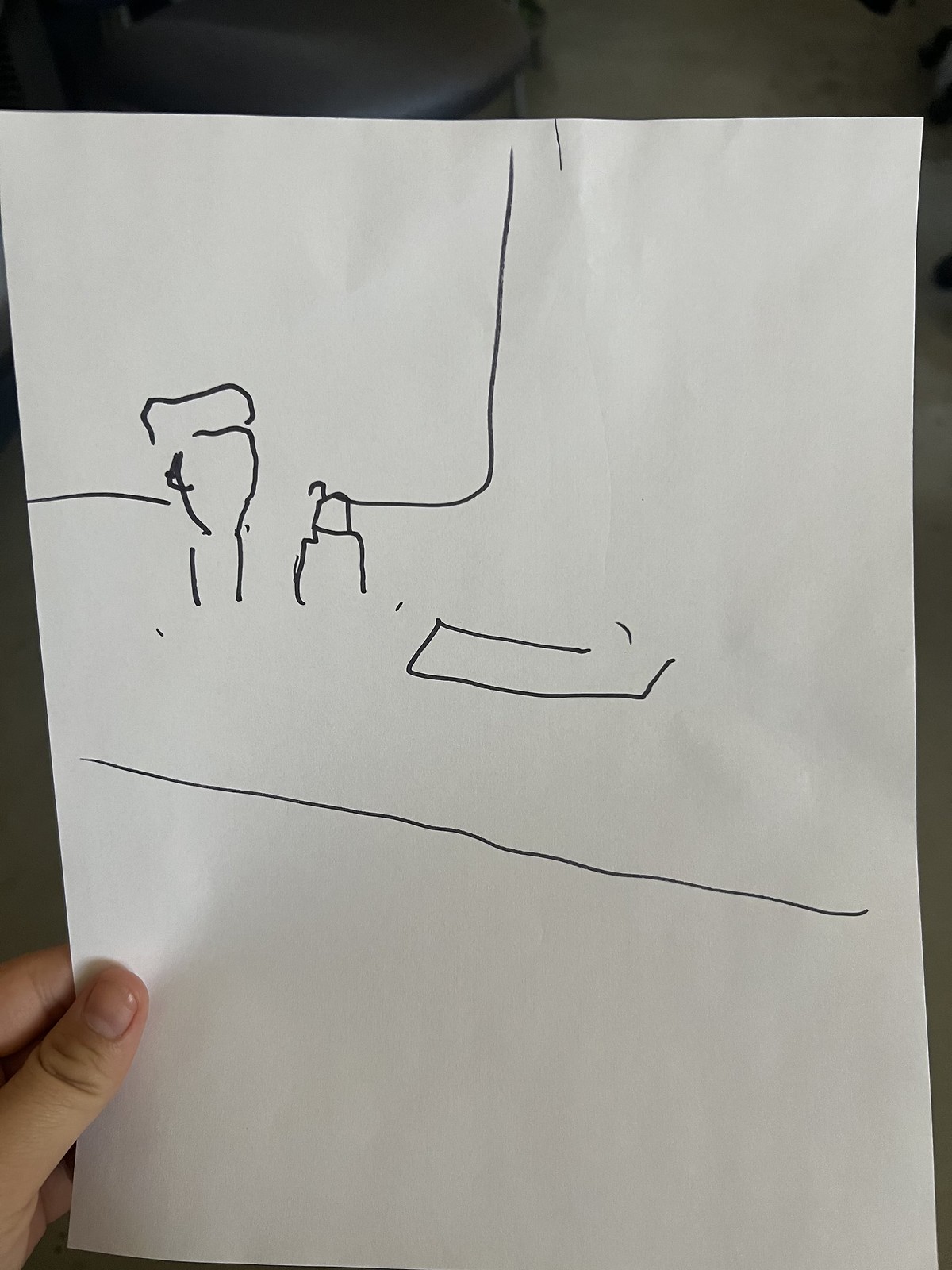In this image, we see a piece of crisp, white paper adorned with a drawing created using black marker. At the bottom left corner, a hand holds the paper, its nails clear and healthy, showcasing the half-moon on the fingernail indicative of good health. The drawing itself is abstract and puzzling. 

A horizontal line stretches across the page from left to right. Above this central line, there is an almost complete rectangle, defined by three sides. To the left of this rectangle, there is an ambiguous shape resembling a rock, nearly square in form with a small square-like feature on top. Further left, a larger object mirrors this shape but differs slightly; it starts with two straight lines at the bottom, then forms an upside-down triangle, topped again by an almost complete rectangle missing its bottom side.

In the background, another horizontal line traverses the entire width of the paper before turning vertically and extending straight up, reaching the middle of the top part of the page. The composition is minimalist and leaves much to interpretation, inviting viewers to ponder its meaning.